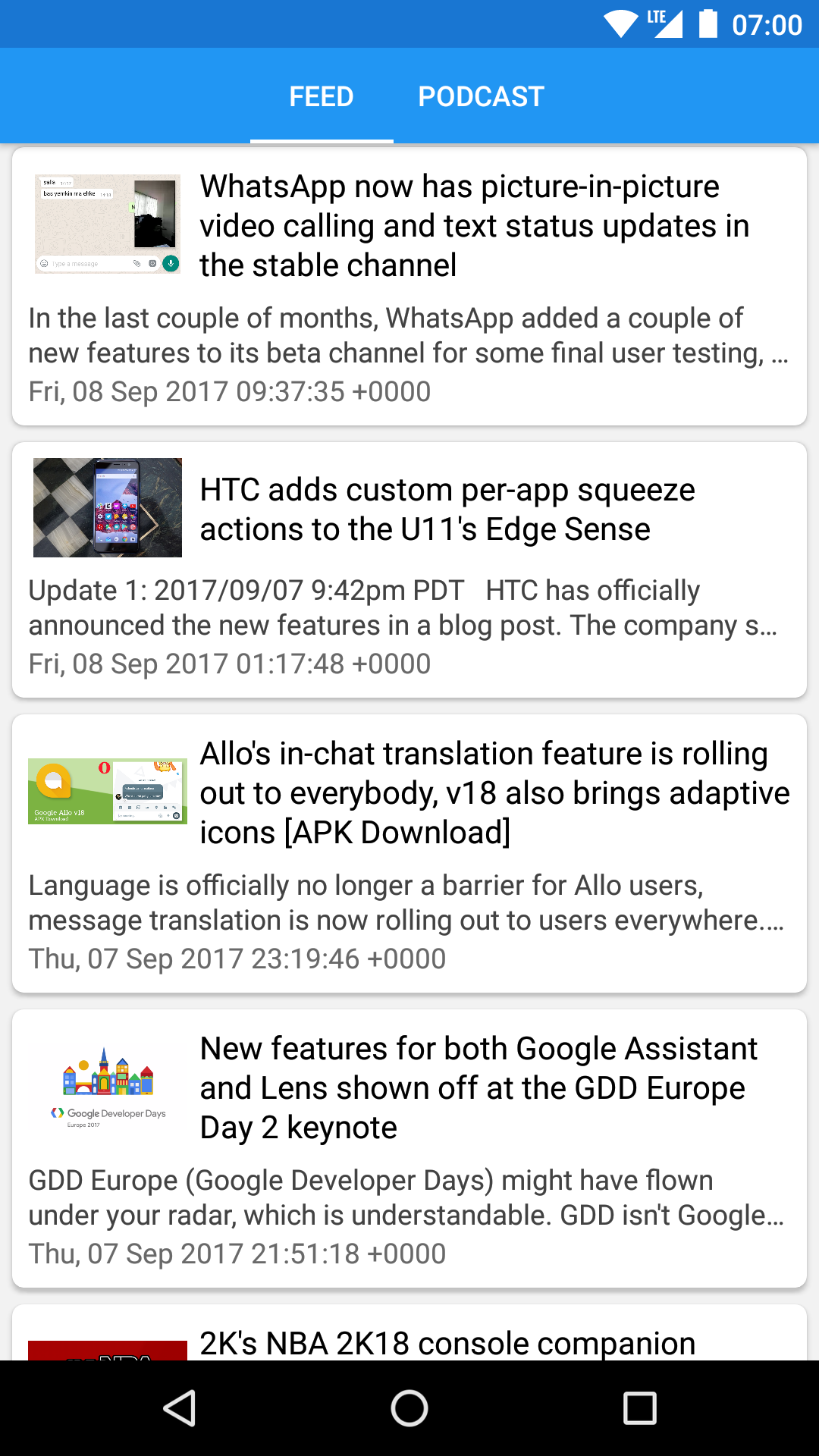A screenshot from a smartphone displays the interface of a content application. At the top of the screen, there are two blue bars. The uppermost bar is a darker blue, while the one immediately below it is a lighter blue. The darker blue bar is slimmer compared to the lighter blue bar. On the top-right corner, the status indicators show the "LTE" signal, a full battery icon, and the time "7:00."

Below this, there is a white line separating the navigation options, with "Feed" on the left and "Podcast" on the right—both labels are in white text. Scrolling down the page, the main content consists of a series of rectangular sections, each featuring a headline and a thumbnail image on the left. The visible headlines include:

1. "WhatsApp now has picture-in-picture video calling and text status updates in the stable channel."
2. "HTC adds custom per-app squeeze actions to the U11's Edge Sense."

The content continues downwards, with a total of five sections visible if the user were to scroll further. However, the lowest section appears partially cut off. At the very bottom of the screen, there is a black bar containing three white icons: an arrow, a circle, and a square, likely representing navigation buttons.